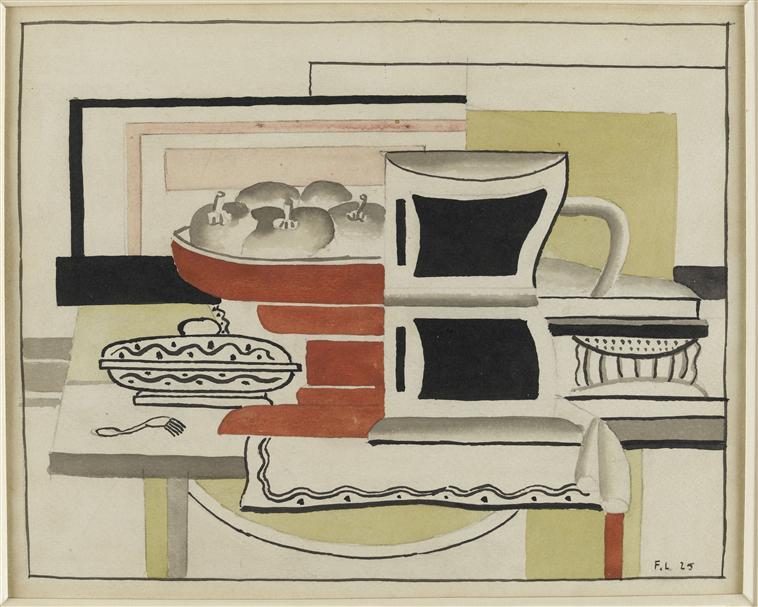The artwork is a mixed-media drawing, combining pencil, marker, and possibly acrylic paint. It centers on a still life composition featuring a red bowl of fruit, predominantly white apples, set on a white table runner adorned with black squiggly lines along the border. To the right of the fruit bowl sits a black and white coffee mug, while to the left, there is a bent fork and an apple pie dish. The setting includes a black and white placemat on a yellow carpet, beneath a table against a backdrop marked by geometric patterns involving black, white, pink, and yellow hues. Additional lines in black and gray weave through the piece, with hints of brown, yellowish-green, and pink faintly visible. In the bottom right corner, the painting is signed with the initials "FL" and dated either February 25th or denoted by the numbers 15 or 19, which are difficult to discern clearly.